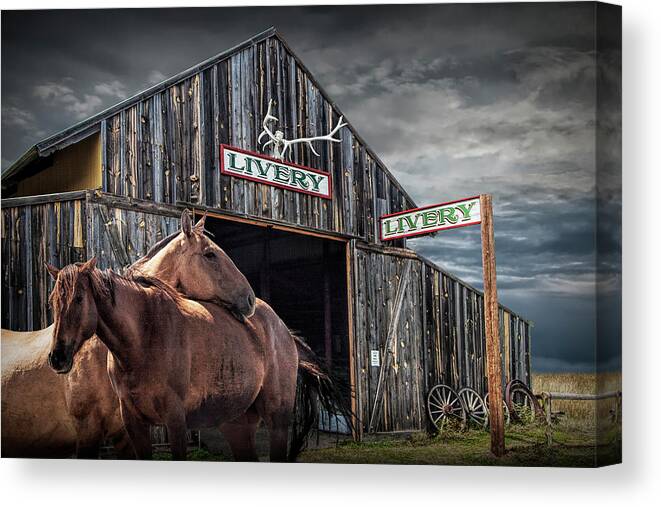The image portrays an old, stylized livery stable crafted from artistically exaggerated wood, giving it a rustic and slightly run-down appearance. The livery stable is prominently adorned with a large stag's head and antlers as its primary advertisement. In the foreground, two brown horses stand close to each other, one resting its head over the back of the other, seemingly seeking comfort as dark, brooding skies loom above, hinting at incoming rain. The livery, with a sign displaying "LIVERY" in green lettering on a white background with a red outline, appears twice: once directly on the barn and again on a wooden post in front of it. Surrounding the stable are numerous spare wagon wheels propped against its exterior, as if waiting to be affixed to carriages. The scene evokes a rural atmosphere with vast open spaces stretching around the stable. Despite the gloomy clouds dominating the sky, a ray of sunlight gently illuminates the horses, adding a touch of warmth to the otherwise somber setting.